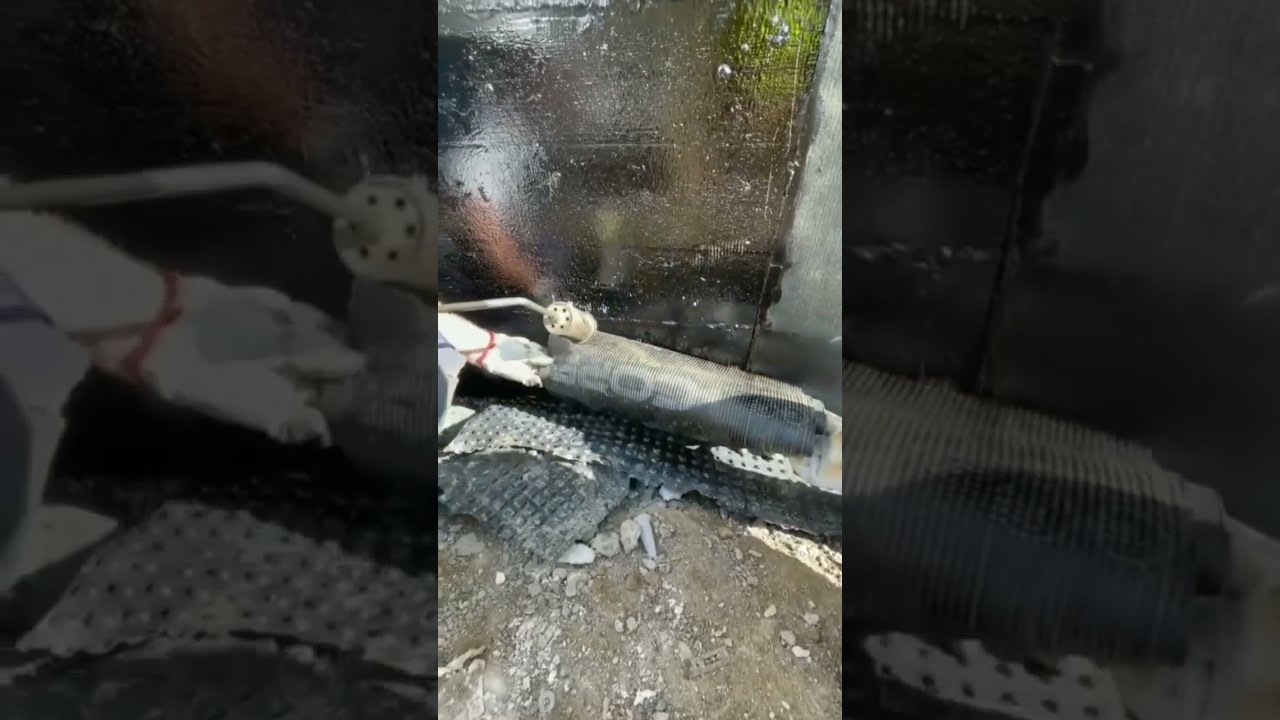The image showcases a rectangular photo divided into three vertical panels. The center panel is brightly lit and in full color, drawing primary focus, while the left and right panels appear darker with an opaque filter effect, seeming like blown-up versions of the central panel's sides. The central image reveals a deteriorated concrete floor and a worn-out cinder block wall featuring various colors, including green on the right, black, and white, possibly from graffiti or peeling paint. This wall has a rough texture with white spotting throughout. On the floor, there are remnants of black matting, torn and rolled up, suggesting an ongoing remodeling project or cleanup of an old basement or garage area. Additional details include a bent metallic pole attached to a cylindrical object, scattered debris, and partial lettering on the floor matting. The surrounding panels provide close-up views of these elements, particularly emphasizing the bent pole, matting holes, and highlighted sections of the damaged wall.